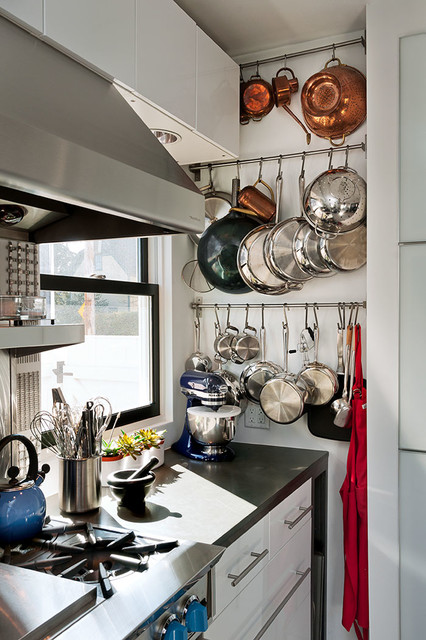This indoor daytime photograph captures a cozy and functional kitchen scene. Dominating the lower left corner is a silver gas stove with a black burner on the bottom right and a blue tea kettle on the back burner. Directly above the stove is a vent hood. The dark gray or black marble countertop extends from the stove to the right, featuring white drawers with silver handles beneath it. In the corner of the countertop near the stove, there's a silver container filled with whisks, spoons, and tongs, accompanied by a small black mortar and pestle. A blue KitchenAid mixer with a silver bowl is positioned in the upper right corner, near three small white pots with plants. Directly above the countertop is a window that lets in daylight, revealing a glimpse of grass outside. To the right, the white wall sports horizontal bars with hooks, supporting an array of hanging pots, pans, and colanders, and a red apron is prominently displayed on the far right hook. The combination of kitchen appliances and organized hanging utensils creates a well-equipped and inviting culinary workspace.